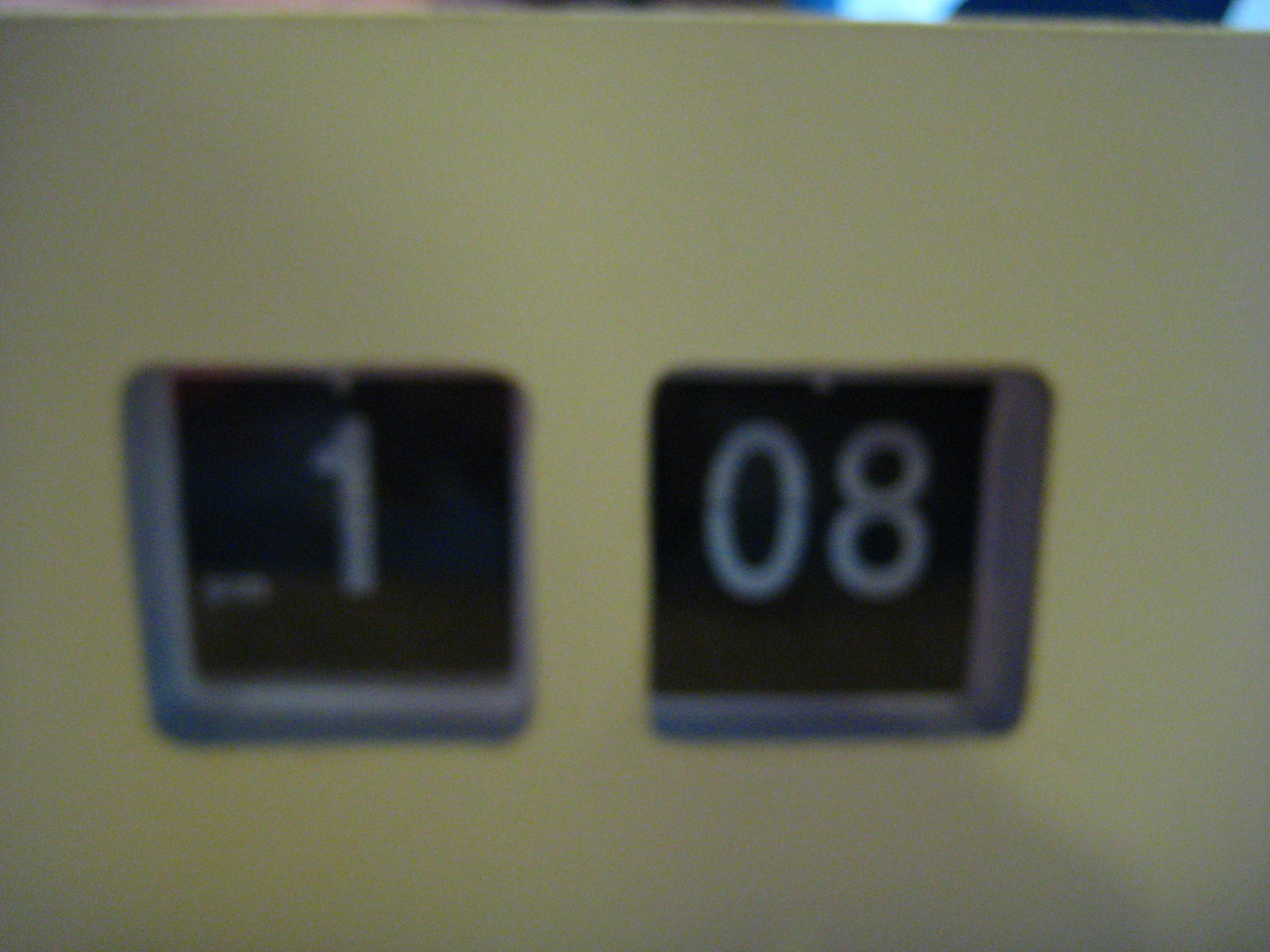A fuzzy, out-of-focus image features a tan-colored, rectangular clock with a simple, minimalist design. The clock face is divided into two distinct sections: the hour display on the left and the minute display on the right, both set against a black background. The left hour window shows the number "1" and is bordered by a thick gray edge on the left and bottom sides, while the right minute window shows "08" with a gray edging on the bottom and right sides. Notably, the top and right of the hour window and the left and top of the minute window lack borders. In the upper right-hand corner, light and dark blue colors blend subtly. The image is shadowed, adding a layer of depth to the scene.